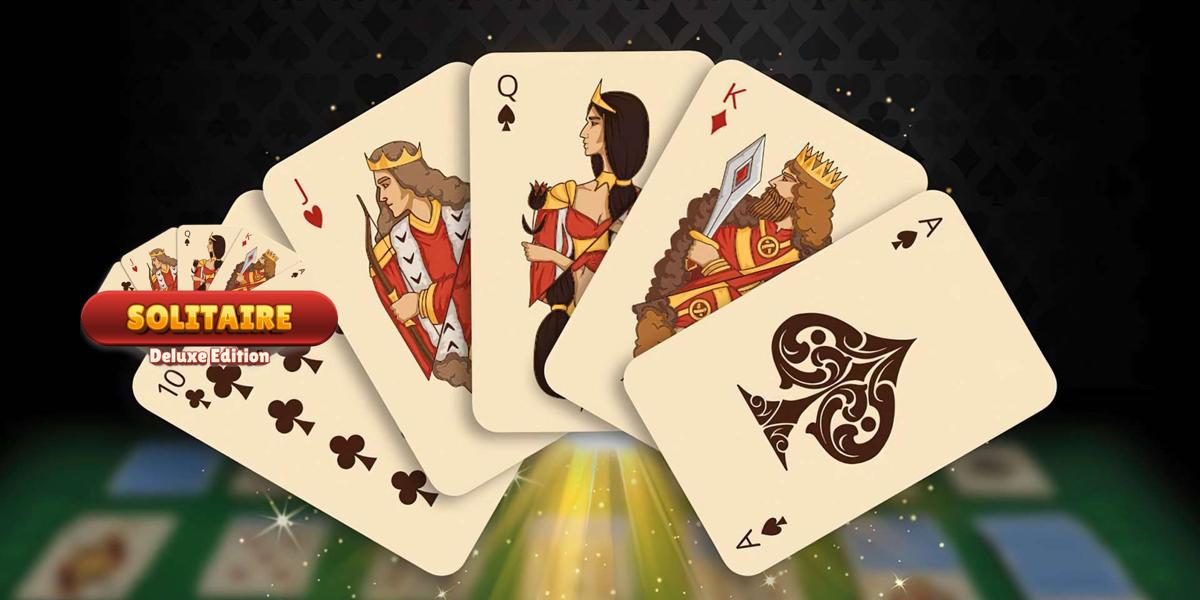This is an advertisement for a video game titled "Solitaire Deluxe Edition." The image is rectangular with a visually striking and detailed composition. In the foreground, prominently displayed, are five large, face-up playing cards: an ace of spades, a king of diamonds, a queen of spades, a jack of hearts, and a ten of clubs. The king and jack sport brown hair, while the queen has black hair; all three figures wear crowns.

To the left, there's a round, red emblem with yellow lettering that reads "Solitaire" and below it, in white with a red outline, "Deluxe Edition." Surrounding the cards are stars and rays of sunlight emanating from the center, adding a radiant effect.

The background features a black wallpaper adorned with spade, diamond, heart, and club patterns, providing a textured backdrop. Below, a green table is partially visible, with cards laying face up and a deck face down to the right, all slightly out of focus to emphasize the central elements.